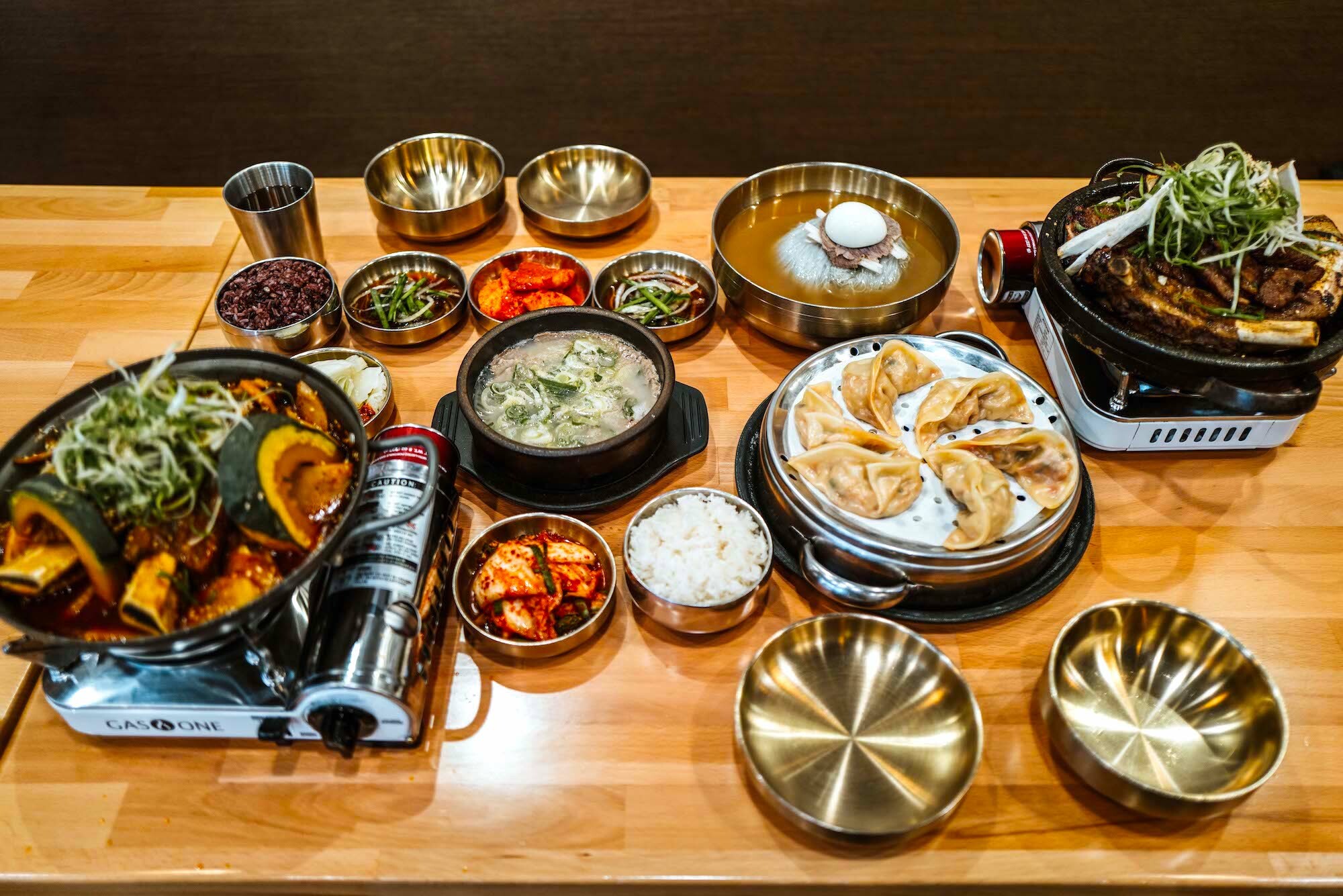The image captures an extensive spread of various foods, all elegantly arranged on a pair of flat, rectangular wooden tables pushed together to form a larger dining area. This scene likely takes place in a restaurant or an eating-dedicated room. The front part of the composite table features multiple brass and stainless steel bowls, some empty and others filled with different kinds of food, including what appears to be green string beans, a silver bowl containing gravy, and another bowl that possibly holds dumplings. In the background, on the left side of the table, a gas stove with an attached canister and a black knob is in use, cooking a squash-filled soup in a black bowl. On the right, another similar stove hosts a bowl filled with what looks like animal ribs. The table setup emphasizes a communal and diverse dining experience, reflecting a variety of dishes prepared and served with care.